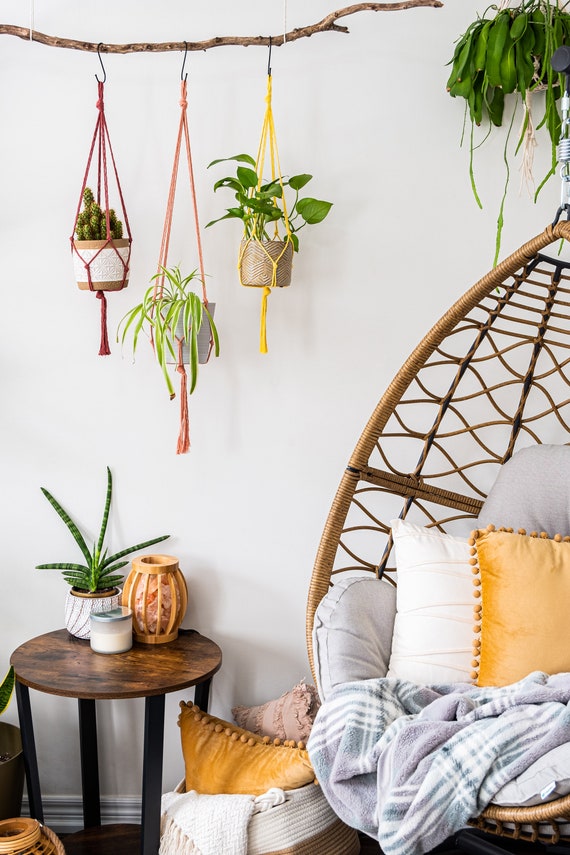This carefully staged photo, seemingly designed for a magazine or blog post, depicts a serene room abundant with houseplants and cozy furnishings, giving off a bohemian vibe. Dominating the right side of the image is a hanging teardrop chair, half-visible, adorned with an inviting array of pillows in yellow, white, and gray, along with a matching gray blanket. To the left of the chair is a basket containing more pillows, including an orange and a dusty pink one.

A small, round wooden table with four black legs stands to the further left, topped with a vase, a small plant, and a white candle. Suspended from the ceiling by a twig are three hanging plants, each in a different color hanger – red, orange, and yellow – adding a touch of whimsy and color to the scene. Additionally, the upper right corner of the image features another hanging houseplant, partially visible. The room's white walls and the earthy tones of the decor create a harmonious and inviting atmosphere, perfect for relaxation.